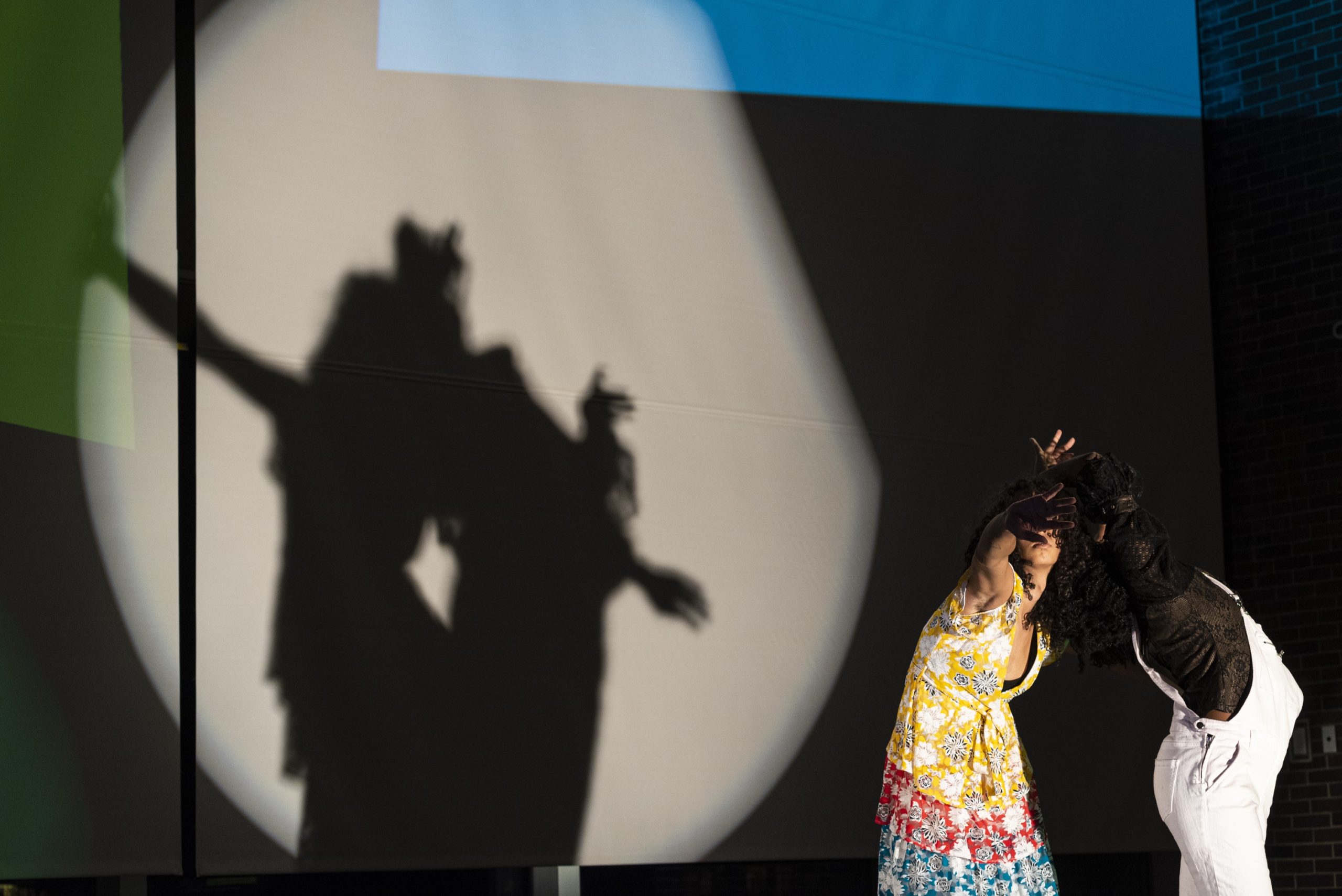The image captures a dramatic stage performance featuring two figures. On the right side of the stage, a person in white overalls and a black shirt stands with their right arm extended upward in a dramatic pose. To their left, a woman with curly brown hair, dressed in a vibrant yellow top and a red, blue, and white floral dress, leans toward them, also raising her right arm. Both figures are illuminated by a spotlight, casting intricate shadows on a beige backdrop that add depth and mystery to the scene. The top of the backdrop features parts of a blue square and a green square, while the rest of the stage remains shrouded in black, highlighting the performers and their captivating silhouettes.